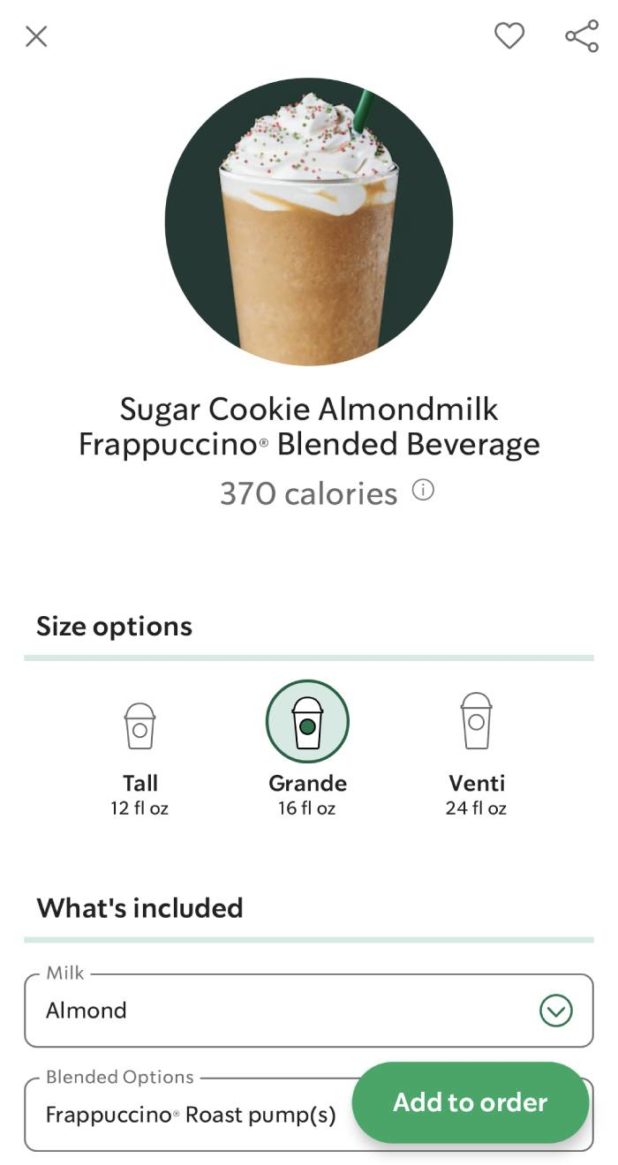The image, captured from the Starbucks app on a smartphone, showcases a delectable Sugar Cookie Almond Milk Frappuccino Blended Beverage. Dominating the top of the screen is a striking black circle featuring a close-up of the fancy coffee drink, characterized by its tan hue. Crowning the beverage is a generous swirl of whipped cream adorned with festive sprinkles, and a straw is seen inserted into the drink. 

The screen indicates the drink's calorie count at 370, accompanied by a heart icon for favoriting the drink, and a share button for forwarding it to others. A small "i" enclosed in a circle is adjacent to the calorie count, presumably offering more detailed nutritional information upon selection.

Size options are listed underneath in a dropdown menu, offering choices of Tall (12 fluid ounces), Grande (16 fluid ounces), and Venti (24 fluid ounces), which are akin to small, medium, and large sizes. The "What's Included?" section elaborates on customizable aspects: milk type, which is currently set to almond milk, and the option to add Frappuccino roast pumps. A prominent "Add to Order" button is superimposed at the bottom, inviting users to finalize their selection.